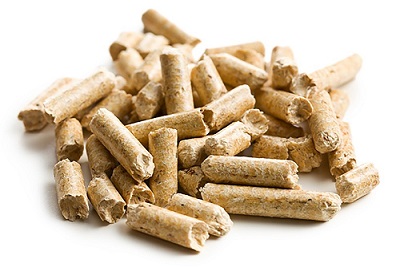The image shows a centrally positioned pile of small, broken, light brown cylindrical pieces against an all-white background. The pieces, which resemble sticks or small cylinders, vary in length with some standing upright and others lying flat. They are densely clustered, making it difficult to count but approximately 40 pieces appear to be present. The material appears to be the same throughout, with some pieces featuring tiny white specks inside, similar to broken crayons. The photo might be an advertisement for a food product, given their crunchy appearance, but the exact nature of the items is unclear. Despite the minimal context, the central focus is this piled collection of uniformly colored, fragmented objects.